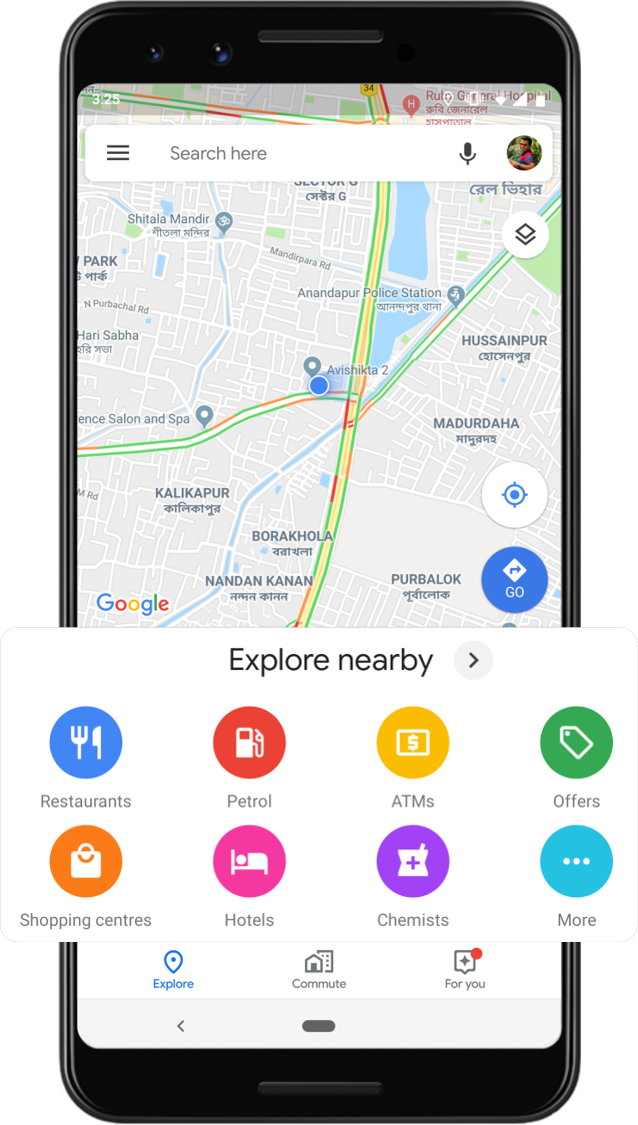The image captures a smartphone with its screen actively displaying the Google Maps application. The map is centered around a location in India, as denoted by place names like "Nandapur Police Station" and other local annotations. A vivid blue dot on the map signifies the user’s current location. Dominating the top of the screen is a white search bar, located in the upper right corner of which is a user profile icon. The icon depicts a male with dark hair, wearing sunglasses and a blue shirt, suggesting it may be the owner of the device.

The map itself features a mix of main roads, smaller roads, and various streets, providing a detailed view of the area. Notably, there is a large lake situated towards the center of the map, and an oval shape visible in the top right-hand corner, likely a park or a sports ground.

Towards the bottom of the screen, there is an "Explore Nearby" section that extends beyond the screen's physical borders, suggesting it provides extensive options for local exploration. This section includes eight clickable icons representing categories like restaurants, petrol stations, chemists, hotels, and more, offering quick access to nearby amenities.